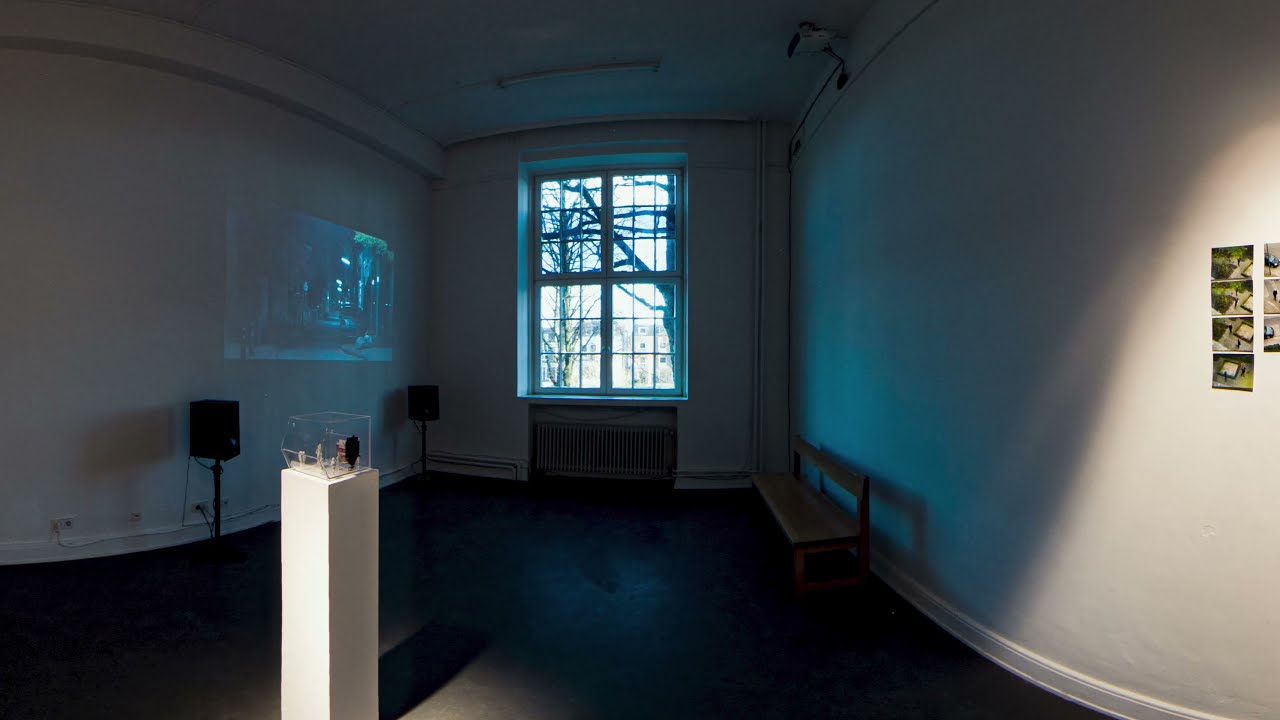The photograph captures an indoor space that seems to be a part of a museum or exhibition room, distorted possibly by a fisheye lens. The room is dimly lit, with light streaming in from a large square window on the far wall, giving a view of a cloudy day and a leafless tree outside. The walls inside are white, featuring a slight curvature on the right. There is a bench along the right wall and eight pictures displayed towards the edge of the photo. On the left side of the room and closer to the window are a couple of cubical black objects, possibly speakers, mounted on vertical stands. In the immediate foreground stands a small white rectangular pillar or platform, showcasing a transparent glass or plastic box containing indistinguishable items, resembling artifacts, that might suggest the room’s function as an exhibition space. A radiator is situated beneath the window, adding to the room's details.